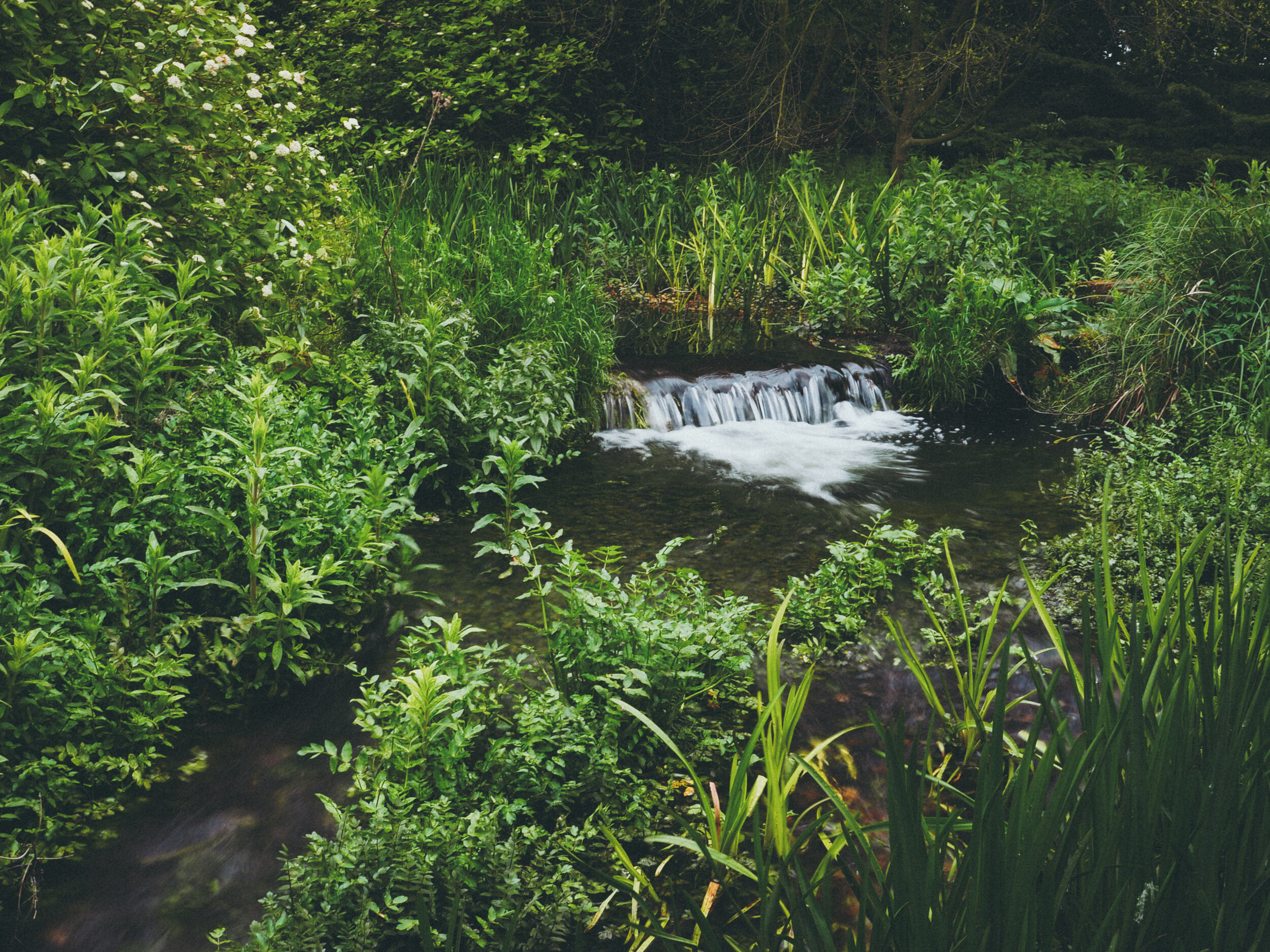This outdoor photograph captures a serene and picturesque scene centered around a small waterfall, no more than a foot high, cascading into a larger pool of water. The waterfall, adorned with white foam at its base, leads into a tranquil stream. The lush green vegetation, comprising wild weeds and various plants, envelops the stream on all sides. The background features several trees with dark green leaves, some of which are felled and moss-covered. To the top left, there are plants blooming with white flowers, adding a touch of delicacy to the verdant landscape. The image exudes a peaceful, natural ambiance, suggestive of a secluded woodland area.